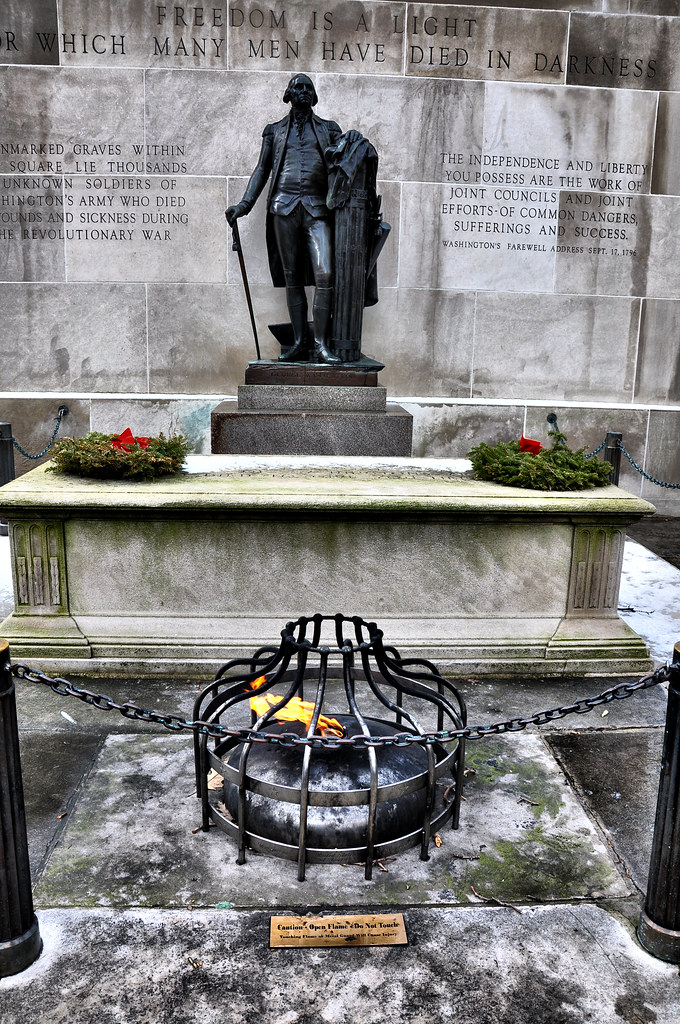The photograph captures a detailed and solemn monument dedicated to George Washington, featuring a realistic black sculpture of him dressed in a jacket and vest. Washington holds a long sword in his right hand, using it as a cane, and his left hand rests on a nearby pillar. He stands on a stone pedestal, backed by a massive gray brick wall that prominently displays the engraved quote, "Freedom is a light for which many men have died in darkness." 

In front of the statue is a small, white coffin-shaped monument encircled by a chain barrier, preventing visitors from crossing. Within this enclosed area, a flame burns brightly inside a little cage-like structure, symbolizing eternal remembrance. Adjacent to the flame, there is a golden plaque and two wreaths placed on either corner of the cement platform. Additional inscriptions flank the left and right sides of George Washington on the wall, further contributing to the poignant atmosphere of this public memorial space set upon weathered tiles.